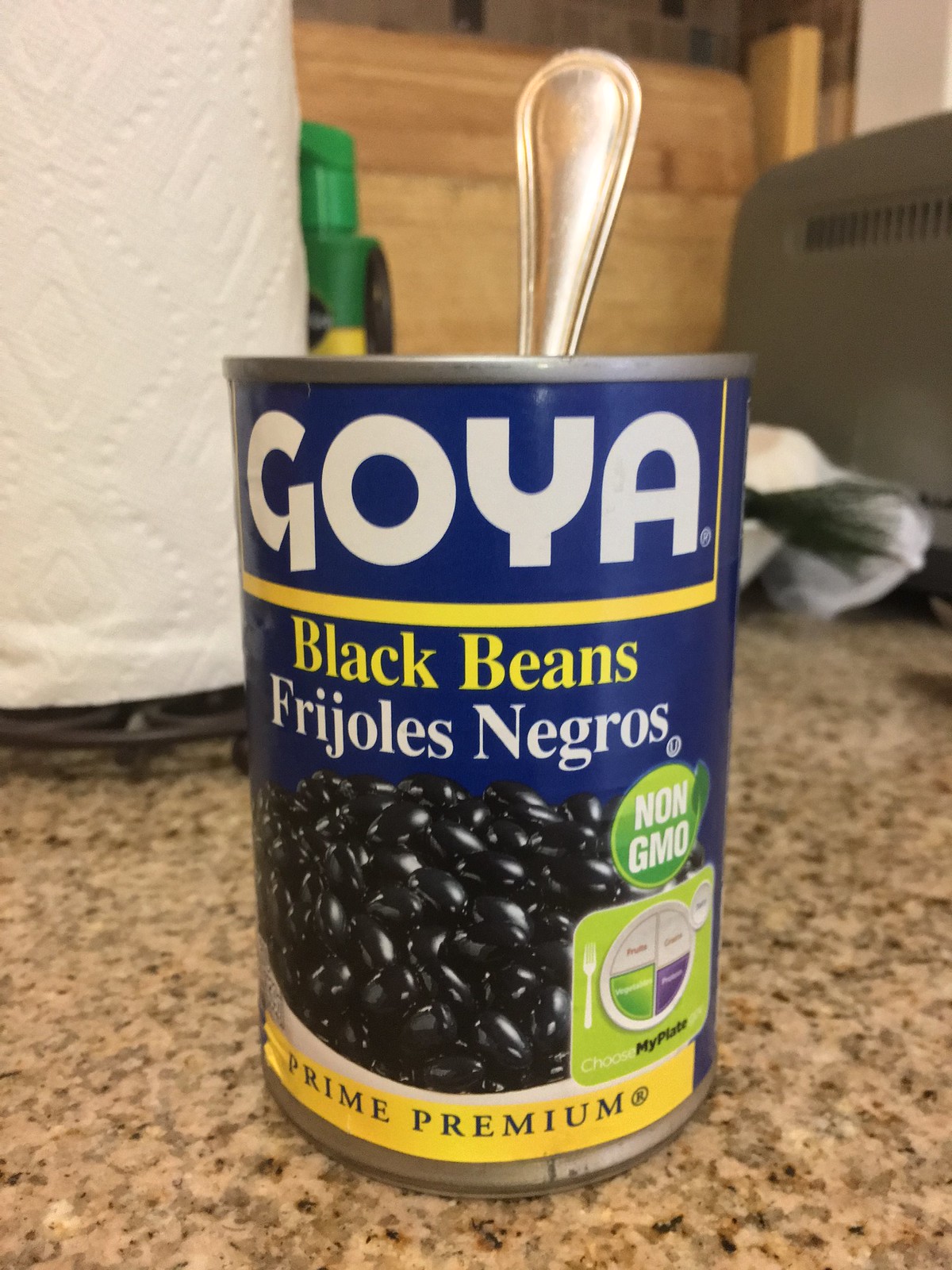A detailed image description capturing the scene:

In this image, the foreground features a smooth granite countertop, characterized by its gray hue interspersed with black and white speckles. Atop the countertop lies a white paper towel, notable for its embedded dots and diamond patterns. To the right of the scene, contrasting white tiles and a gray appliance with an inbuilt vent can be seen in the background. A wooden texture is visible close to the paper towel, adding warmth to the setting.

Towards the left side of the image, a plastic bag is partially protruding, hinting at some activity or usage. Adjacent to this is a container bearing colors black, red, and yellow, which appears to resemble a soil package.

Prominently positioned in the foreground is a blue can of Goya black beans, adorned with the brand's white text "Goya." Below the brand name, a white and yellow stripe accompanies the words "Black Beans" in yellow, and the Spanish translation "Frijoles Negros" in white text. Scattered black beans lie artistically near the can, adding texture to the scene. The lower label indicates "Prime Period" with a non-GMO stamp on the top right of the can.

To the right of the beans, there is a dietary reference plate, labeled "ChooseMyPlate," with sections denoted at the top left, top right, and bottom segments, symbolizing food group divisions. A fork is placed to the left of the plate, completing the organized layout. An additional small icon appears at the top right, possibly representing a side item or drink.

All these elements together create a diverse and detailed kitchen-oriented scene.